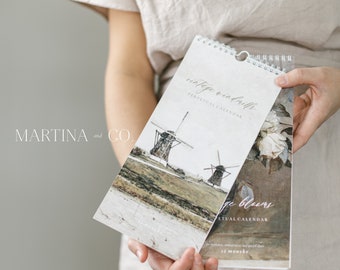The photograph features a partial view of a woman, shown from the waist down, wearing a light gray tunic-style dress. She is holding two narrow, spiral-bound notebooks or calendars, outstretched in front of her with both hands. The top notebook prominently displays an image of two windmills, while the other is mostly obscured but possibly features a floral scene. The color scheme of the image is gray-toned, with the background consisting of a gray wall that occupies the left third of the frame. In white lettering on the background to the left, the text reads "Martina and Co." The overall composition is minimalist, focusing primarily on the person's hands and the items they are holding.